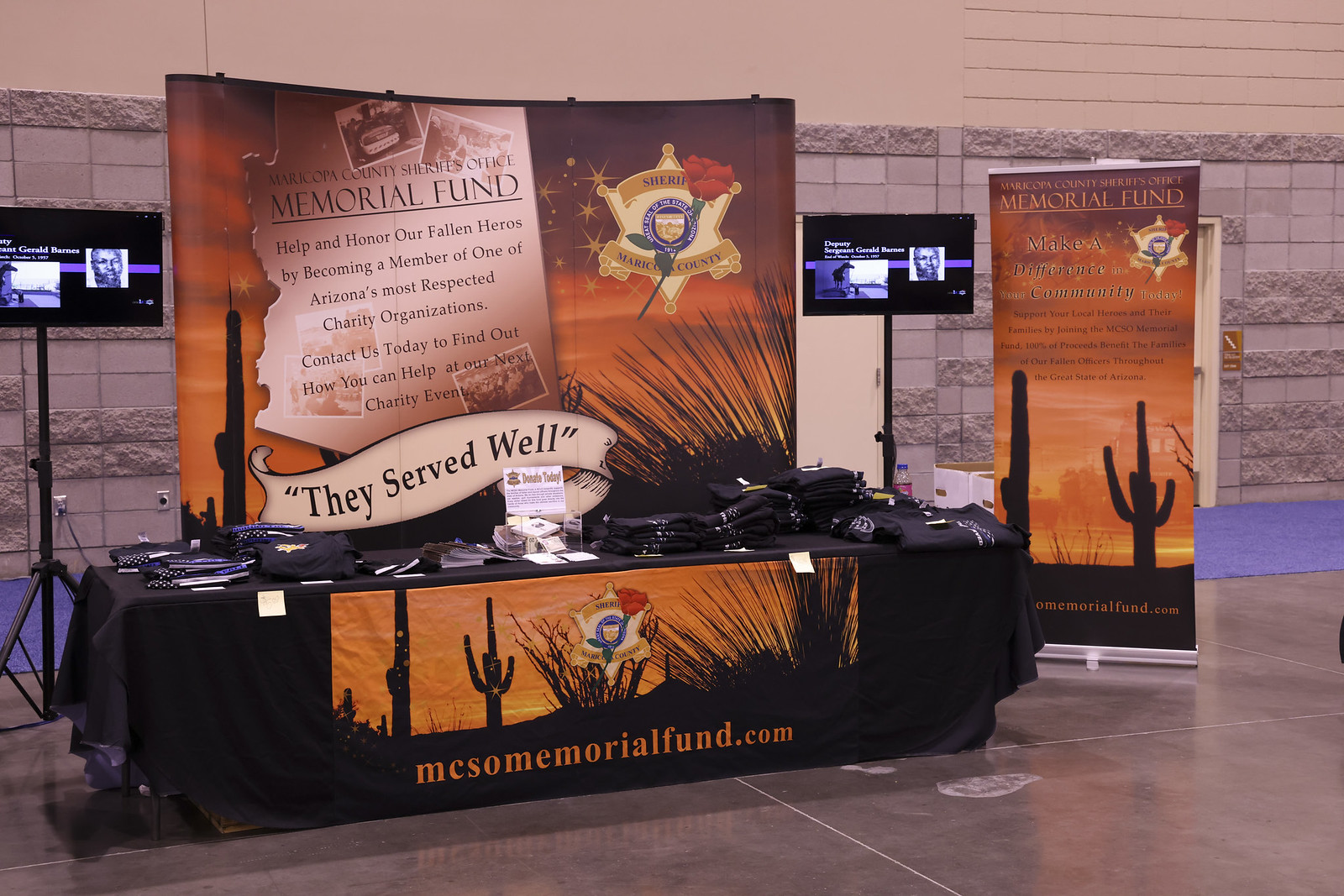The image shows a detailed setup of a memorial fundraiser for fallen heroes of Arizona. Central to the scene is a black tablecloth-covered counter extending from the lower left to the center-right, decorated with an image of an Arizona desert scene at sunset, complete with cacti and the state flag against a golden sky. Across the front of the tablecloth is the URL "MCsomeMemorialFund.com". Displayed on the table are various items including black shirts, jerseys, and bags.

Behind the table, a prominent large sign reads "Memorial Fund" against a brown, possibly sky backdrop. The sign includes text urging people to "Help and honor our fallen heroes by becoming a member of one of Arizona’s most respected charity organizations." Below this statement, the words "they served well" are also visible. 

Nearby, another rectangular sign also bears the "Memorial Fund" branding. Additionally, two video screens positioned behind the table display identical images on black screens featuring some blue graphic. The background setting of the image consists of granite gray walls and a solid gray tiled floor, with lighting providing clear visibility of all these elements.